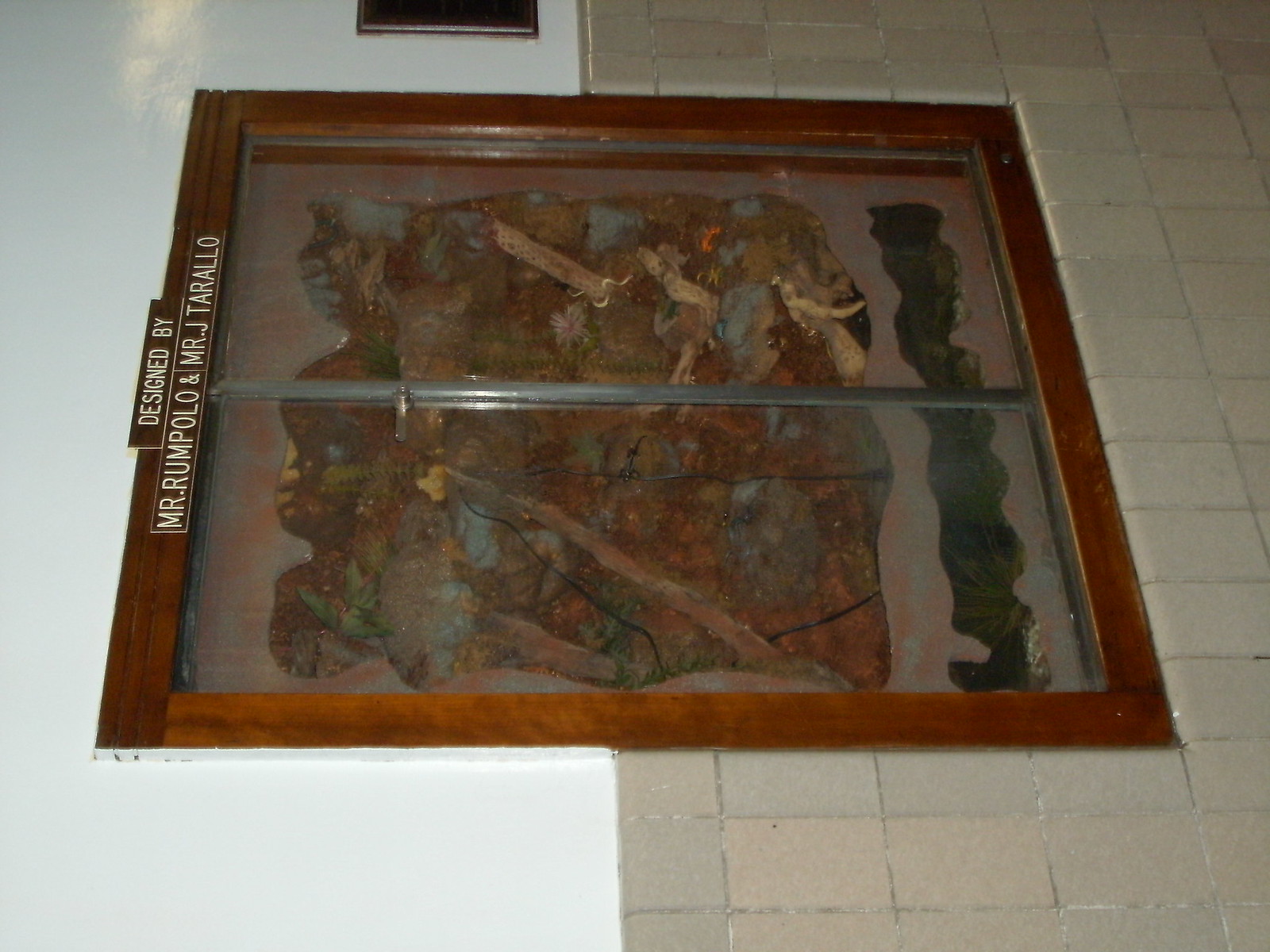This photograph, taken indoors, possibly in a church or school, shows a piece of artwork integrated into a wall. The image is displayed sideways, requiring rotation to view correctly. The art display is set within a wooden frame and protected by a glass cover, which appears to be split into two panes. The wall behind the artwork is white on the upper half and tiled with beige tiles on the bottom half, reminiscent of school tiling. The artwork itself features a jungle or fairyland scene with green, brown, and beige tones. At the top of the display, which is on the left side due to the orientation of the photo, a plaque reads "Designed by Mr. Rampolo and Mr. J. Tarallo" in white letters. The scene includes a motif of green plants and evokes an underground or mythical atmosphere.